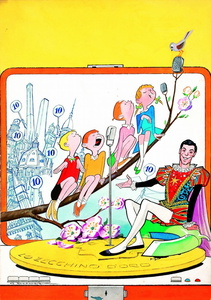The image depicts a whimsical and vibrant cartoon scene with a Renaissance-inspired theme. At the bottom-right, a man dressed in royal garb, complete with puffy shoulders, white stockings, black shoes, and a red garment, sits on a green cushion atop a large yellow, coin-like disc. His right hand is outstretched towards the left side of the image. Surrounding him, a predominantly yellow background is accented by a rectangular lunchbox-shaped item with a red band across the bottom.

Extending from the left, a large, curved branch stretches towards the man's hand. Perched along this branch are four children, each dressed in colorful attire: a girl with pigtail braids wearing a blue dress and green bows, a red-headed girl in a pink shirt and green shorts, a boy with red hair in a yellow sweater and orange shoes, and another boy with blonde hair in a red shirt, black pants, and yellow shoes. Atop the branch, a white bird looks down at the children, seemingly participating in their song. Below the children, another branch adorned with flowers protrudes from the left side of the image.

In the background, a white board with a red border and a topsy-turvy cityscape add an additional layer of intrigue to the scene. The overall composition suggests an enchanting, musical moment designed to entertain, featuring a blend of playful and formally attired characters in a fantastical setting.